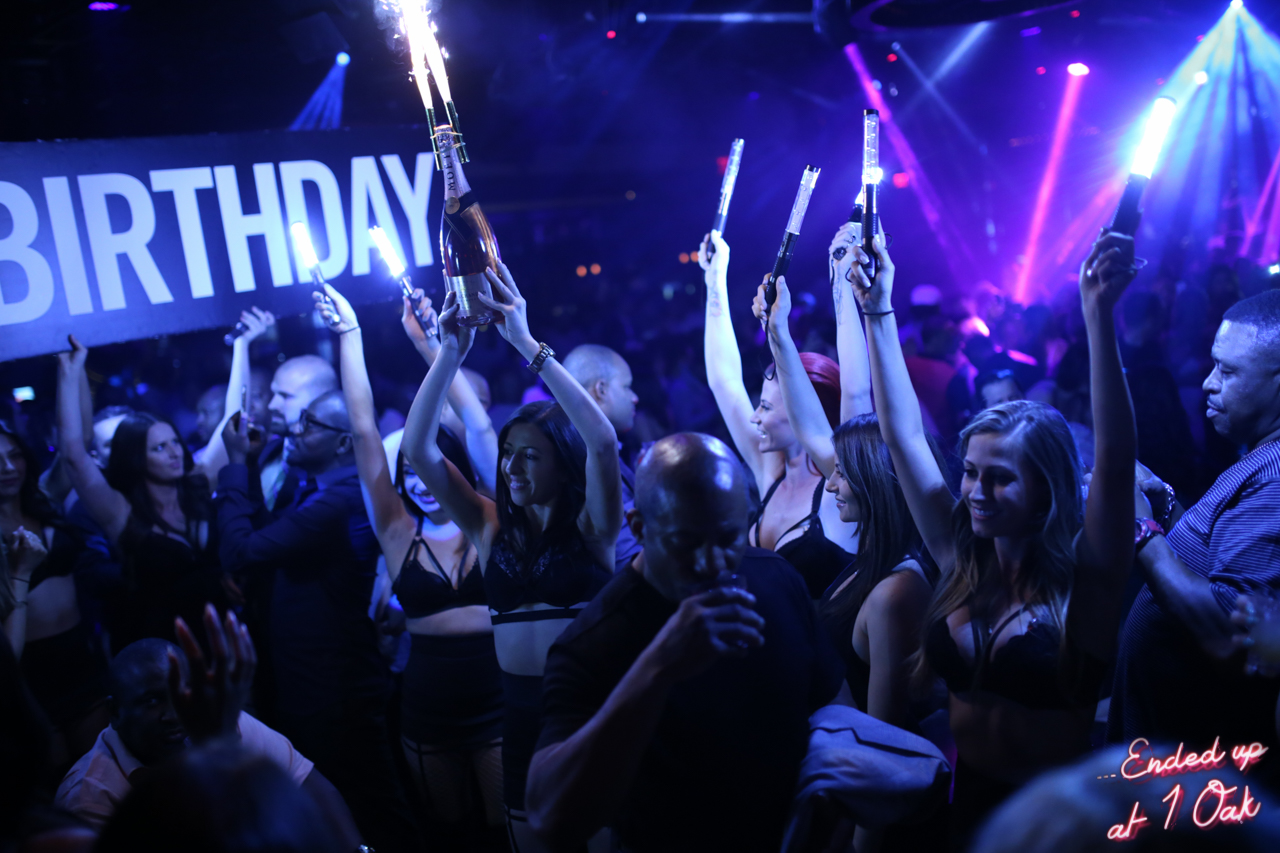The vibrant photograph captures a bustling birthday celebration at a nightclub or dance club. A crowd of men and women, many with their hands raised high, holding various party ornaments and lights, are seen smiling, laughing, and dancing. Spotlights and colorful lights—blue, pink, and purple—illuminate the background, enhancing the festive atmosphere. A prominent woman in the center holds a champagne bottle aloft, which is spectacularly shooting out flames or sparkles. To the left side of the image, a large blue banner with "birthday" written in white text is held up, likely by several people. While the women are dressed in fancy attire, the men appear to be in regular shirts. In the lower right-hand corner, neon cursive text reads, "Ended up at One Oak," marking the location of this exuberant celebration.